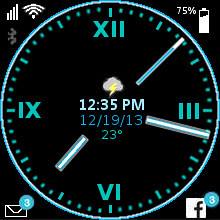The image depicts the interface of an electronic clock, possibly from a smartphone app. The clock face features only the primary Roman numerals (XII, III, VI, IX) while the other hour markers are absent. At the center, there is an icon of a small cloud with a lightning bolt, indicating stormy weather. Directly below the cloud symbol, the time is displayed as 12:35 p.m., accompanied by the date "12/19/13" and a temperature reading of 23 degrees. 

The clock itself is a round blue dial with white hands. The minute and hour hands indicate a time around 7:17, and the second hand is positioned slightly past the 1 o'clock mark. This entire display is set against a black square background. 

In addition, several indicators are present on the frame: 
- The upper right corner shows a battery icon with a 75% charge.
- The upper left corner displays typical phone status icons, including signal bars and internet connectivity.
- The bottom left corner features an envelope icon with a blue circle showing the number 3, indicating new messages.
- The bottom right corner shows a Facebook icon with a similar blue circle and the number 3, indicating notifications.